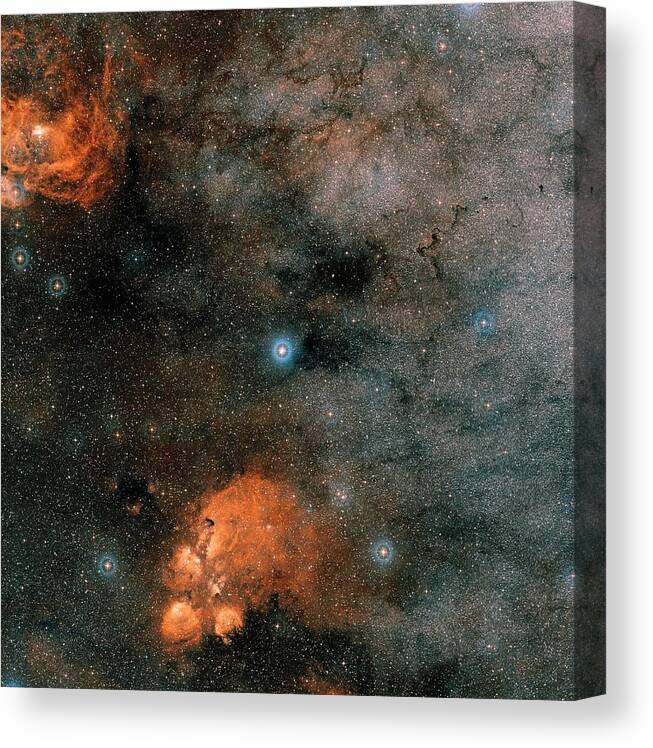The image is a high-quality, professional painting or canvas print depicting an outer space scene. The background is primarily black with sparkly, star-like specks scattered throughout. There are distinct orange and reddish-orange clouds, one in the top left corner and one in the bottom center, which may represent gaseous formations or nebulas. These clouds add a warm tint to the otherwise dark expanse. The painting also features several larger, round white and blue spots that may represent prominent stars or planets. These are distributed across the image, with one particularly bright spot positioned centrally, surrounded by a blue halo. The right side of the image shows the thick border of the canvas, providing depth to the artwork. Light pink, light blue, and gray clouds are subtly painted against the dark sky, adding texture and depth. The entire piece has an ethereal, almost mystical quality, evoking the vastness and complexity of the cosmos.